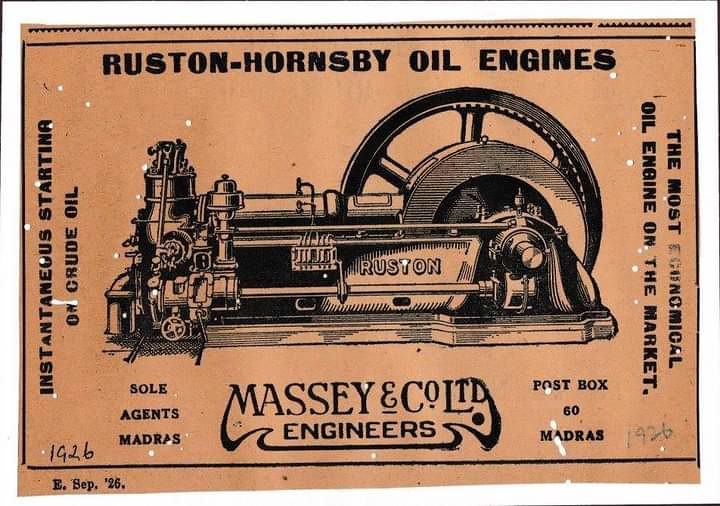The vintage advertisement features an early 1900s Ruston Hornsby oil engine on a light orange background with a landscape orientation. The headline at the top reads "Ruston Hornsby Oil Engines" in bold black print. Centrally, there's a detailed black line art illustration of an old Ruston engine, complete with a prominent crank wheel, suggesting it might be a steam engine. Vertically descending on the left side of the illustration, the text reads, "Instantaneous Starting on Crude Oil," while the right side, flipped in the opposite direction, states, "The Most Economical Oil Engine on the Market." At the bottom center, beneath the engine illustration, is the logo for Massey & Co. Ltd. Engineers, framed by Art Nouveau flourishes. To the right of the logo, it's noted that they are the "Sole Agents Madras" and "Post Box 60 Madras." In the bottom left corner, there's a small, handwritten inscription reading "1926," followed by "ESEP 26." The overall style charmingly captures the era's print advertising aesthetics.